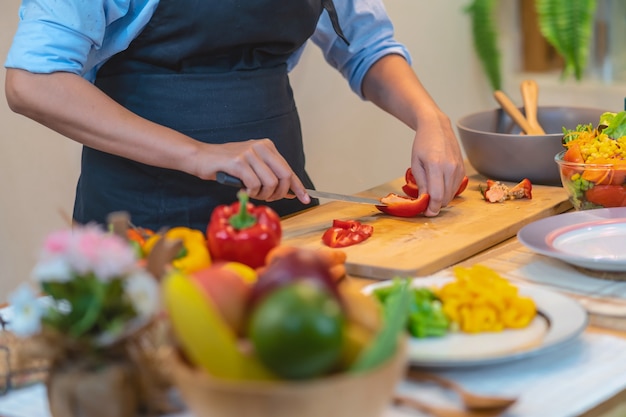In a bustling kitchen, a chef, identifiable only by her midsection and arms, is engrossed in the meticulous task of chopping a vibrant red bell pepper on an oak cutting board. She is dressed in a dark blue apron over a rolled-up blue shirt. Her left hand holds the bell pepper steady while she navigates the knife sideways, risking a precarious cut. The cutting board already holds an array of red pepper seeds. Surrounding her workspace are various bowls and plates, filled to the brim with a kaleidoscope of vegetables—yellow, green, and purple peppers, as well as an assortment of indistinguishable produce. A gray bowl with spoons and a salad bowl containing lettuce, carrots, and corn are nestled among the culinary chaos. The foreground features a basket teeming with whole fruits and vegetables, partially obscured by a soft blur that adds depth to the image. A potted white flower sits to the left of the basket, slightly out of focus, enhancing the scene's vibrant yet cluttered ambiance. The only sharply focused elements of the photograph are the chef's torso, the cutting board, and the red pepper in the midst of being cut, emphasizing the intimate moment of preparation amid the vibrant disarray.